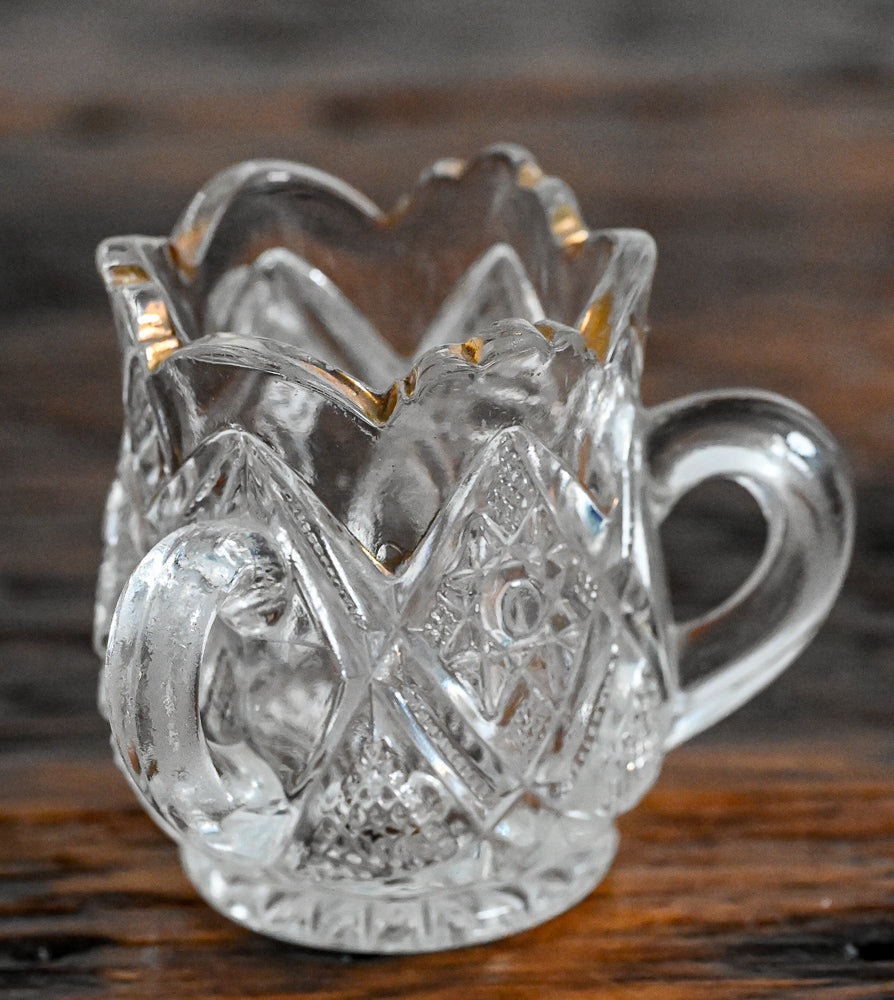This photograph features a clear, ornate glass cup, reminiscent of a piece from a vintage collection. The cup is artistically shaped like a bulb of a flower, possibly a rose, with a bottom that tapers inwards and a wavy, petal-like rim adorned with gold lining. The gold detailing appears worn, suggesting frequent use or age. The cup is embellished with intricate engravings, including diamond and flower shapes, contributing to its elegant design. It has two thick handles, each with small openings that barely fit a finger or two. The glass rests on a dark cherry wood surface, with the background blurred, emphasizing the cup's detailed craftsmanship.